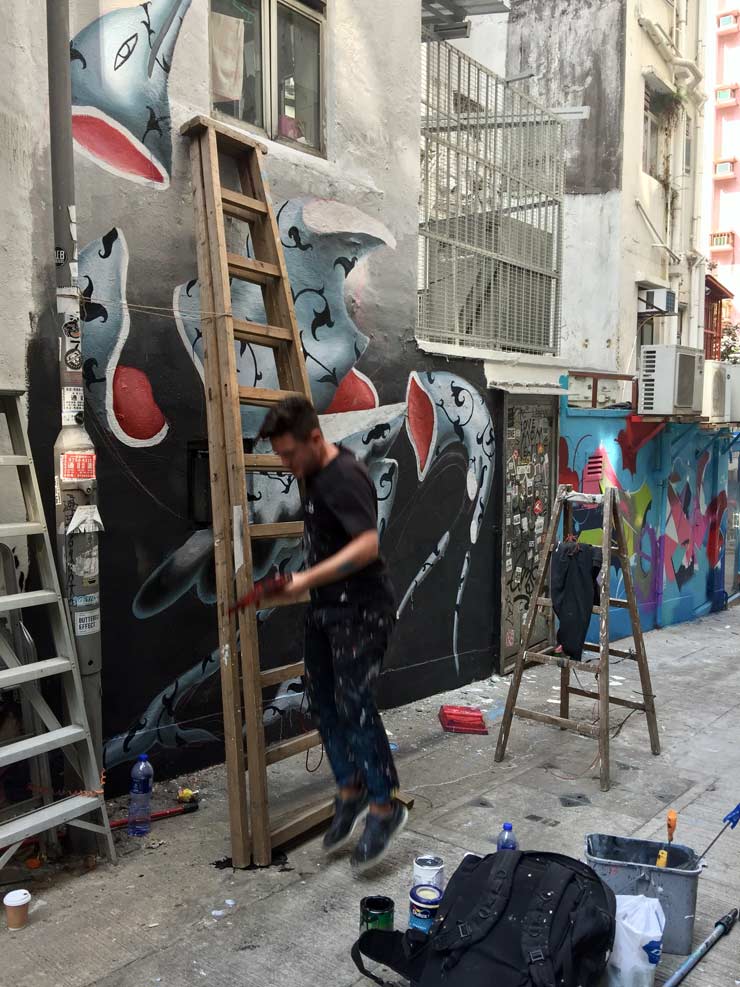In this image, a graffiti artist is captured in motion, either jumping off or onto a brown wooden ladder that is propped, though folded, against a wall. The blurry nature of the photo accentuates his movement. He is wearing a black shirt and dark, paint-stained pants, suggesting he's actively working on the mural. The mural is a vibrant mix of black, blue, and red, depicting abstract shapes that resemble broken fish or shark fins. The scene is set in an alley, with the wall of the building dominating the left side of the picture and getting narrower to the right. Surrounding him are his painting supplies, including a black backpack, paint cans, a bucket with brushes, a trash can, a plastic bag, a water bottle, and a small cup of coffee. The well-maintained alley features numerous air conditioners, and in the upper right, one can see additional buildings in the background, indicating it may be early evening.